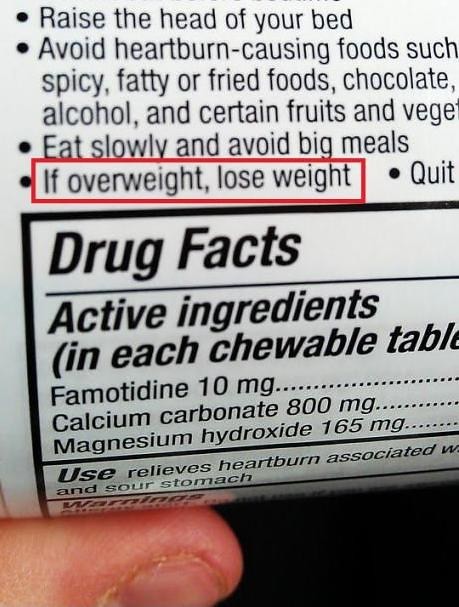This is a close-up photo of a white label with black text on a medication product, held by someone's left hand, with their thumb partially visible against a black background. The label features instructions and information, some of which are partially cut off in the image. At the top, there are four bullet points with health advice:
1. Raise the head of your bed.
2. Avoid heartburn-causing foods such as spicy, fatty, or fried foods, chocolate, alcohol, and certain fruits and vegetables.
3. Eat slowly and avoid big meals.
4. (Enclosed in a red box) If overweight, lose weight.

There is also a partially visible fifth bullet point which starts with "quit," but the rest is cut off. Below these instructions, the label has a section titled "Drug Facts," listing active ingredients per chewable tablet: Famotidine 10 mg, Calcium Carbonate 800 mg, and Magnesium Hydroxide 165 mg. Another section labeled "use" mentions it relieves heartburn and sour stomach, and there's also a "warning" section that cannot be completely read.